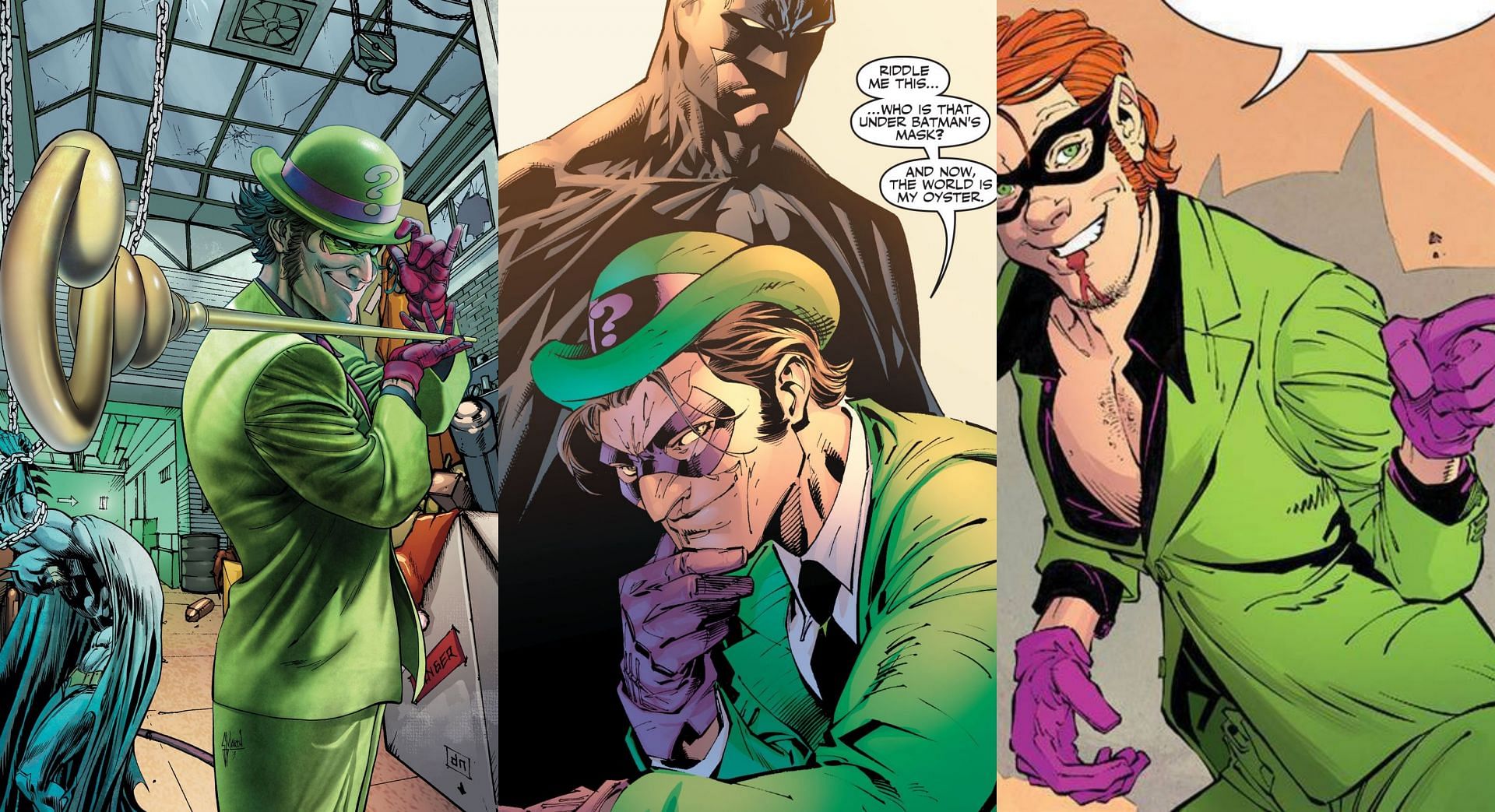The image is a three-panel comic book page featuring the Riddler from Batman. In the first panel, the Riddler is depicted as a large figure resembling a leprechaun, complete with a green suit, a green bowler hat, long sideburns, and fuzzy hair. He is holding a mammoth cane over his shoulder and tipping his hat with a grin. The background features a gray ceiling with hooks, pulleys, chains, and overturned items, suggesting a room used for battles or torture.

In the middle panel, the Riddler is shown in a close-up, grinning and holding his chin. A speech bubble next to him reads, "Riddle me this, who is that under Batman's mask? And now the world is my oyster." Batman, or possibly a representation of him, is seen standing behind the Riddler, adding intrigue to the scene.

In the final panel, the Riddler appears without his hat, a smile on his face, and blood dripping from his bottom lip. He is wearing a black shirt under his green jacket, with red hair, purple gloves, and a black mask. He is pointing and grinning, concluding the series of images with an air of triumph.